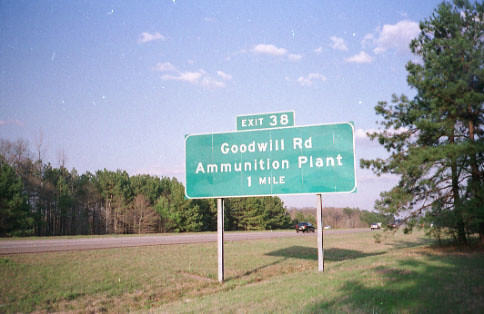This photograph captures the scenic side of a highway, featuring a prominent green highway sign with white lettering and a green trim. The sign displays "Exit 38" on a smaller, elevated section, and "Goodwill Road, RD" in larger letters underneath. Additionally, it indicates "One Plant, One Mile" below the road name. The sign is situated on a grassy embankment that slopes gently into a ditch. In the backdrop, lush trees line both sides of the highway, enhancing the natural setting. Several cars are visible in the distance, traveling along the road, suggesting a sense of motion and activity, although no people are present in the scene. The sky above is a bright, cheerful blue, dotted with fluffy white clouds, adding to the overall cheerful and tranquil atmosphere of the photograph.